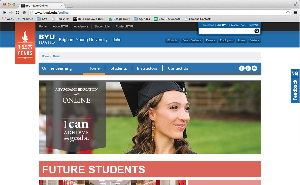This image depicts an open web browser displaying a pixelated webpage of BYU University. Due to the low resolution, most text and details are unreadable. However, "BYU" and "ICANN Future Students" are legible. At the center of the page is a photograph of a woman in a graduation cap and gown, with light skin, brown hair, and set against a green grassy background. A gray ribbon overlaying the photo displays the text "ICANN." Below the image, a darker peach-colored strip features "Future Students" written in white. The top of the webpage includes a navigation strip with "BYU" clearly visible, though the remaining text is too pixelated to decipher. The color palette of the image includes shades of green, black, brown, pink, blue, terracotta, white, gray, and yellow.